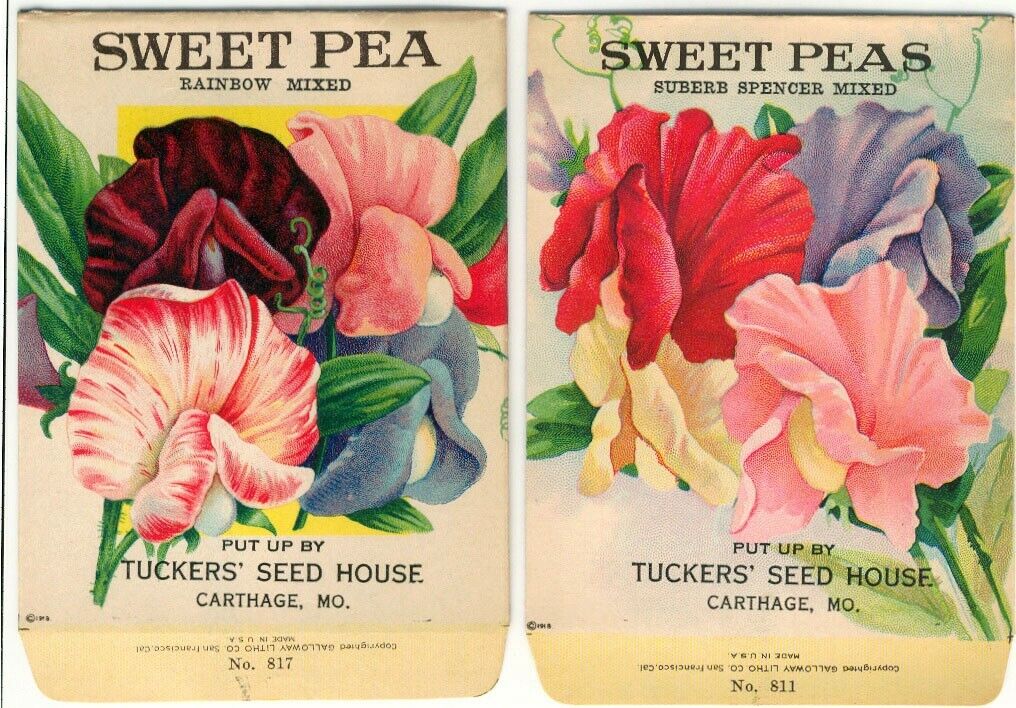The image features two packets of sweet pea seeds side by side, each showcasing vibrant blooms on their respective covers. 

On the left, the packet displays an array of bold-colored flowers, including a striking pink and white striped flower, a deep purplish-red one, a solid pink blossom, and a delicate light blue flower. The top of the packet bears the name "Put up by Tucker Seed House, Carthage, Missouri," with the identifier "No. 817" inscribed at the bottom.

On the right, the second packet presents a different selection of sweet pea blossoms: a singular yellow flower, a light pink bloom, a soft blue flower, and a deep pink one. This packet is marked with the identifier "No. 811" at the bottom.